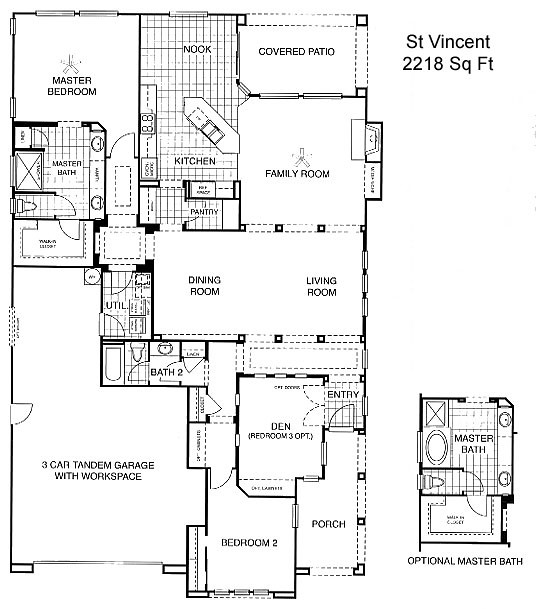This black-and-white illustration depicts a detailed architectural blueprint of a home named "St. Vincent," boasting 2,218 square feet. In the top-right corner, the title “St. Vincent, 2218 square feet” is prominently displayed. The primary layout of the blueprint features the following rooms and spaces:

- **Top-left corner:** Master Bedroom
- **Left side, moving right:** Nook, Covered Patio
- **Left side, moving further right:** Master Bath, Kitchen, Family Room
- **Top-right:** Walk-in Pantry, Dining Room, Living Room
- **Below Dining Room:** Utility Room
- **Below Utility Room:** Bath Two

**Lower left corner:**
- **Three Car Tandem Garage with Workspace**
- **Den/Bedroom Three (Optional)**
- **Entry Area**

**Lower center-right:**
- **Bedroom Two**
- **Below Bedroom Two:** Porch

Adjacent to the main blueprint on the right side, a smaller inset illustrates an optional Master Bath configuration, labeled prominently with "Master Bath" in the center and "Walk-in Closet" underneath.

The layout meticulously organizes each functional space, offering a comprehensive overview of the home design, emphasizing the spacious and versatile living areas.